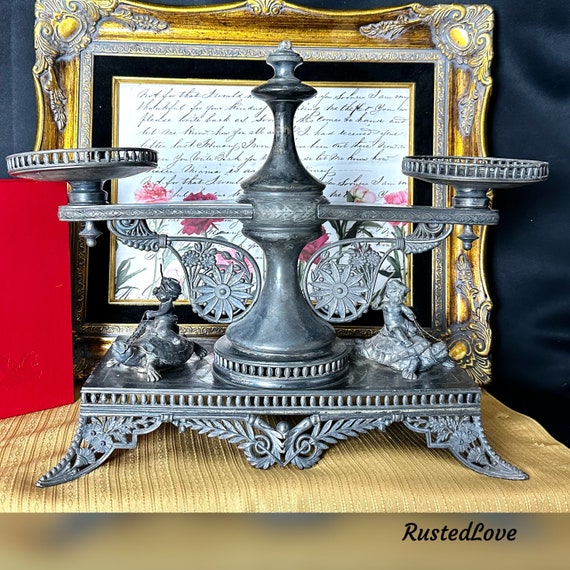This close-up image captures an intricate vintage metal centerpiece or serving piece, prominently featuring a beautifully ornate scale or lamp. The centerpiece boasts a carved base adorned with elaborate scrolls and leaves, transitioning into a silver structure with two finely detailed figures of children riding turtles on either side. Each arm of the scale extends into a circular metal plate, topped with a round, intricately carved finial. The focal piece rests on a tan, striped fabric with delicate weaving patterns, placed atop a fabric-covered chair. Behind the centerpiece, there is a tarnished gold ornate picture frame, enclosing a French drawing or framed document with elegant cursive writing and delicate pink flowers. The image exudes an antique charm, capturing the appeal for vintage enthusiasts. At the bottom of the image, the watermark "Rusted Love" can be seen in a flowing cursive font.